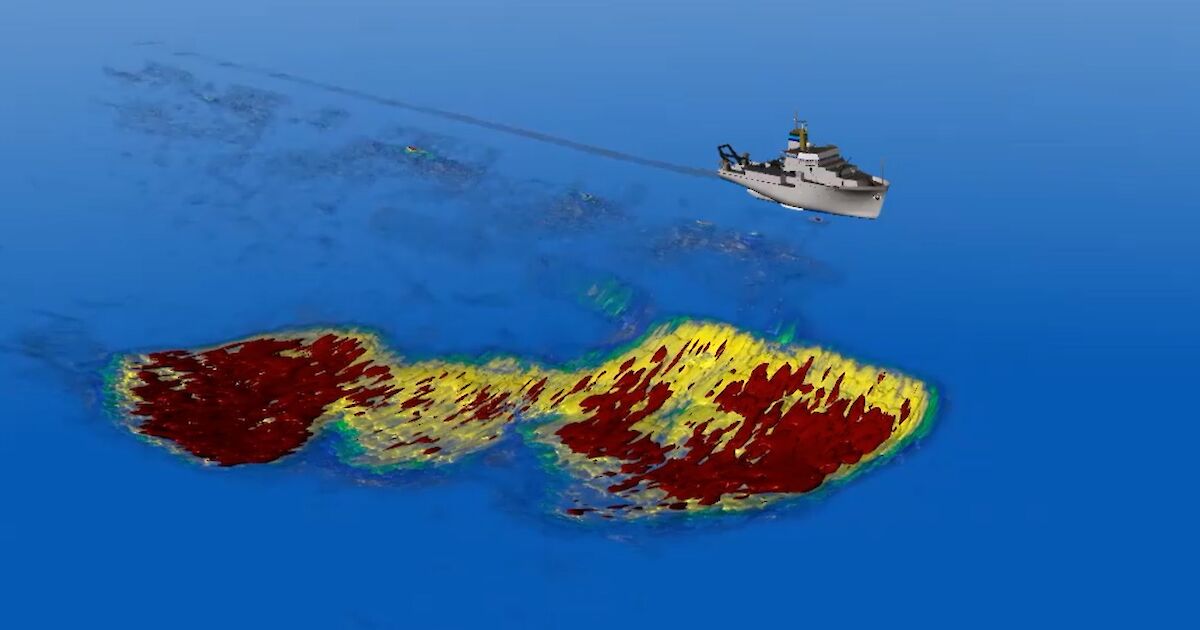The image depicts a computer-generated, polygonal-style representation of a large fishing boat floating on the ocean. The digital artwork has an old or poorly made appearance, characterized by a combination of 3D modeling and painted textures. The boat is primarily silver with some gold accents and piping extending from the top, giving it an industrial look. The vessel features a towering superstructure that rises three or four stories high at the front, with a flat area at the back where fishing nets would be cast.

Surrounding the boat, the ocean is depicted in a deep blue hue, adding to the impression of depth. Beneath the boat, a dark red and yellow mass is visible, resembling a radar image used to detect a large school of fish. This colored splash beneath the water is about three times the size of the boat itself, lending a surreal quality to the scene. Additionally, shadows suggestive of rocks or land formations are visible below the ocean surface, yet these elements don't quite align with the proportions and perspective of the overall image. The digital artwork's combination of 3D modeling and painted elements contributes to its aged and somewhat disjointed aesthetic.